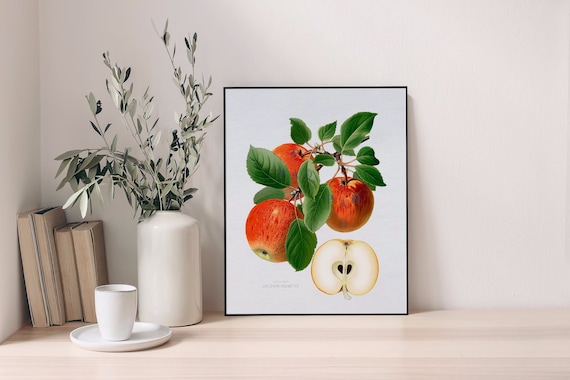The photograph captures a serene still life arrangement set against a plain white background. Central to the composition is a light wood grain table located in the corner of a room. Resting on the left side of the table are four books with their pages facing outward, leaning against the wall. In the foreground, a pristine white saucer holds an empty matching cup. Positioned directly behind this setup is a white vase adorned with long, elegant olive branches. To the right of the vase, a detailed botanical painting of apples catches the eye. The artwork showcases three connected red apples with leaves, accompanied by a meticulously sliced apple half revealing its seeds. The overall setting evokes a sense of tranquility and attention to detail, displaying various homey elements harmoniously.